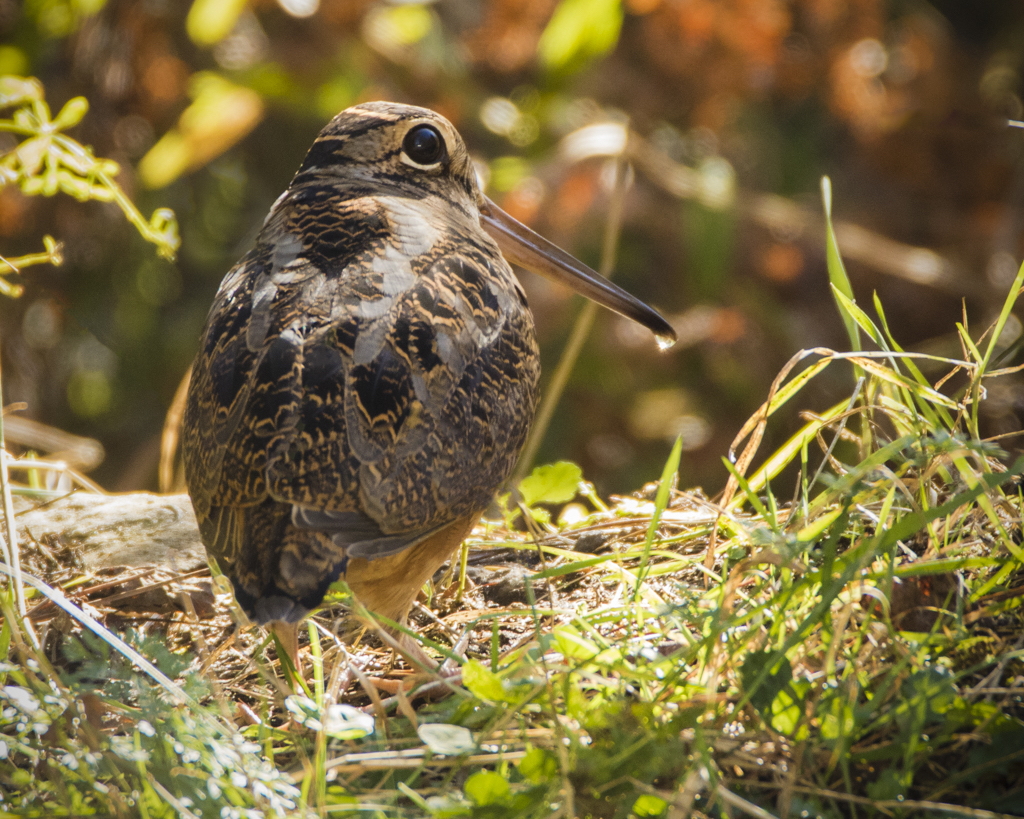In this image, a rotund bird with a striking appearance stands prominently against a natural backdrop. The bird's feathers display a unique mix of black and brown, each feather bordered with a touch of yellow. It has a distinctive long black beak with a delicate water droplet hanging from its tip. Captured in profile, you can see the bird's dark eye and the intricate details of its head and body. The sun bathes the bird and the surrounding area in warm light, highlighting the green clover and grass on which it stands. This grass is interspersed with dirt patches and thicker green leaves, creating a vibrant ground cover. In the blurred background, leaves ranging from green to reddish-orange and scattered sticks enhance the natural setting, suggesting a location rich in greenery, possibly near some trees and shrubs. The bird is positioned slightly off-center to the left, allowing a view of the surrounding environment. Its feet, slightly lighter in color than its feathers, stand out clearly against the green and brown earth beneath.